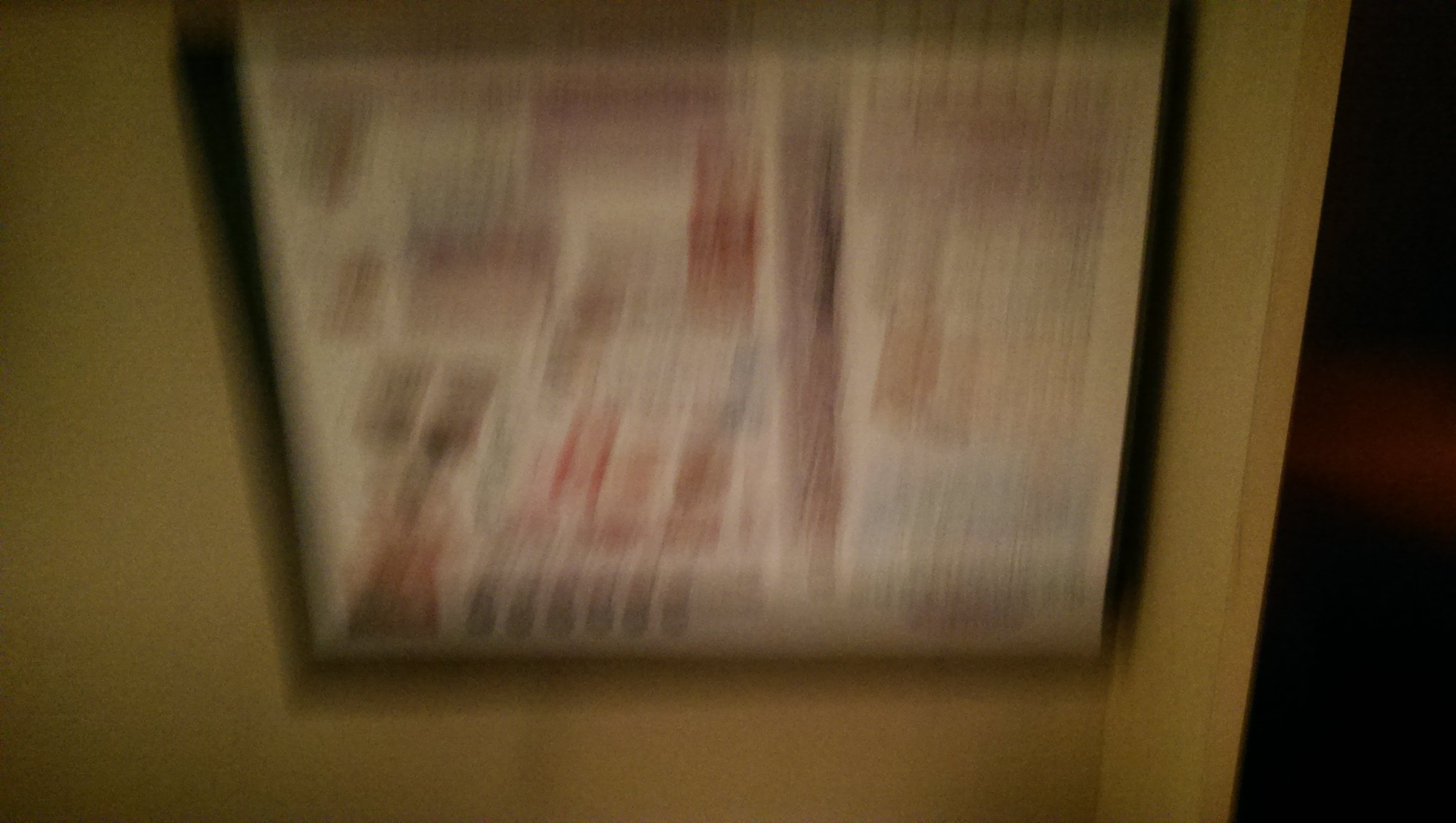The image depicts a very blurry photo of a white poster or menu framed in black, hanging on a yellowish wall with dark, indistinct background areas. The poster measures about four feet by four feet and is structured with various shapes, mainly squares and rectangles, and sections of writing interspersed with pictures. The lower left corner of the frame contains what appears to be six circles. The right side of the image includes a black void or doorway with hints of red. The blurriness suggests that the camera was moving when the photo was taken, rendering the text and images largely indiscernible.